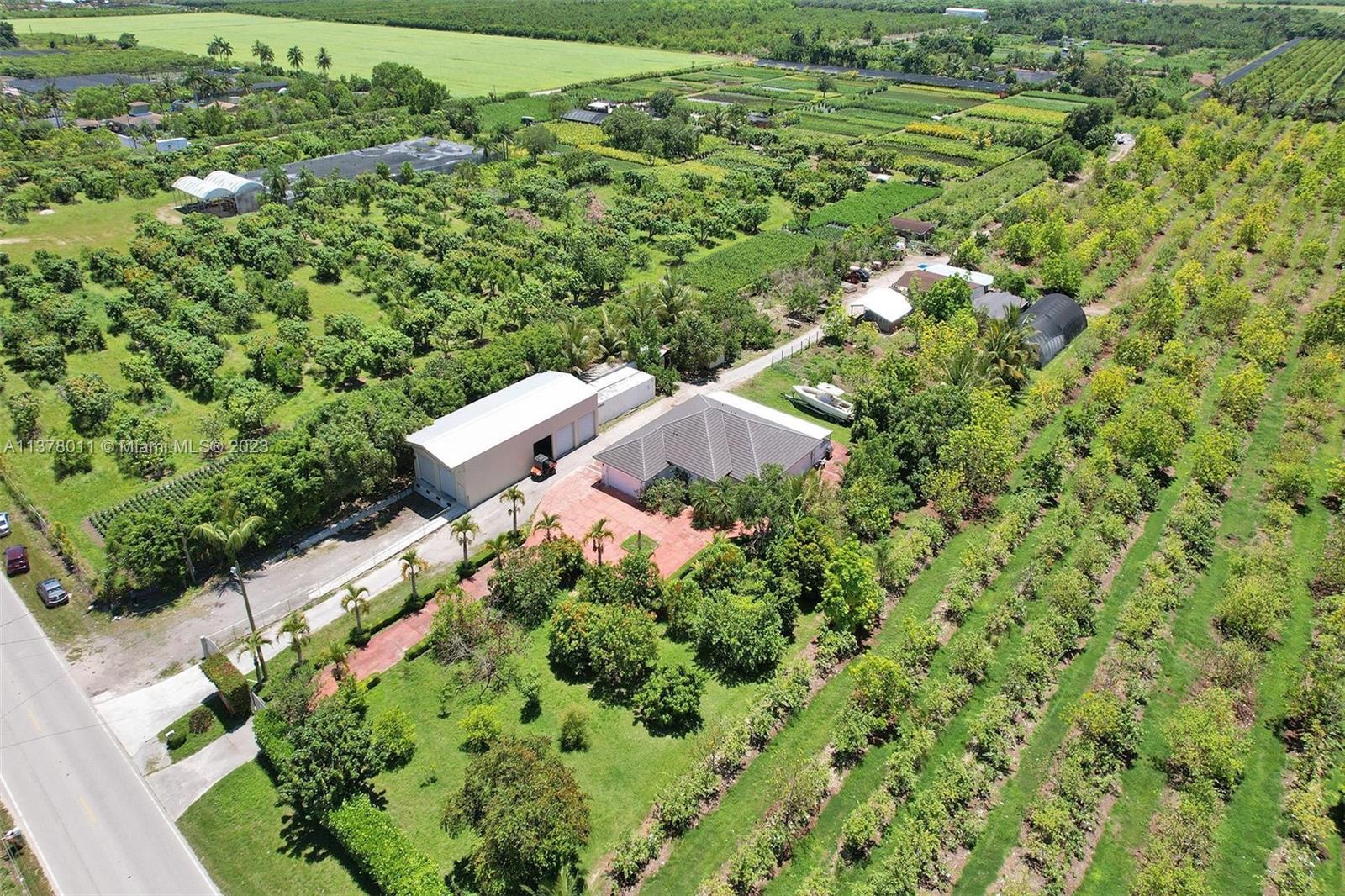This aerial image captures an expansive landscape encompassing several acres of lush, green land. The foreground features a verdant field, densely populated with various trees. Scattered across this area are numerous businesses, identifiable by their sizable white buildings, which resemble large warehouses. Adjacent to these structures sits another substantial facility, characterized by its square shape. A highway runs through the scene, with a few cars parked on the grassy verge. Extending beyond the immediate foreground, the photograph reveals a vast, open field dominated by a continuous expanse of green grass, stretching towards the horizon.